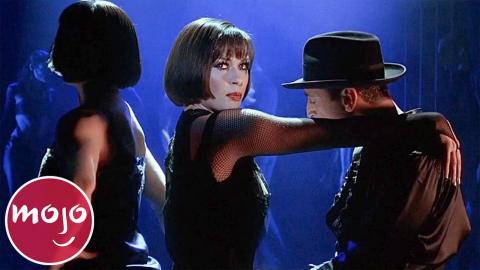This is a detailed thumbnail from a WatchMojo YouTube video, capturing a scene from the movie "Chicago." In the forefront, we see Catherine Zeta-Jones placing her hands on the shoulders of a man wearing a black shirt and a fedora, who is looking down. To the left of her is another woman with the same bob cut hairstyle, dressed in a black outfit. Both women have their backs to each other, and the woman on the right is gazing towards the camera. The background is shaded in dark blue and purple hues, adding a dramatic effect that partially obscures other characters. The WatchMojo logo is prominently situated in the bottom left corner, with the distinctive red circle, white trim, and the word "Mojo" written in white letters. The "O.J.O." in the logo is stylized to resemble a face with eyes and a smile.